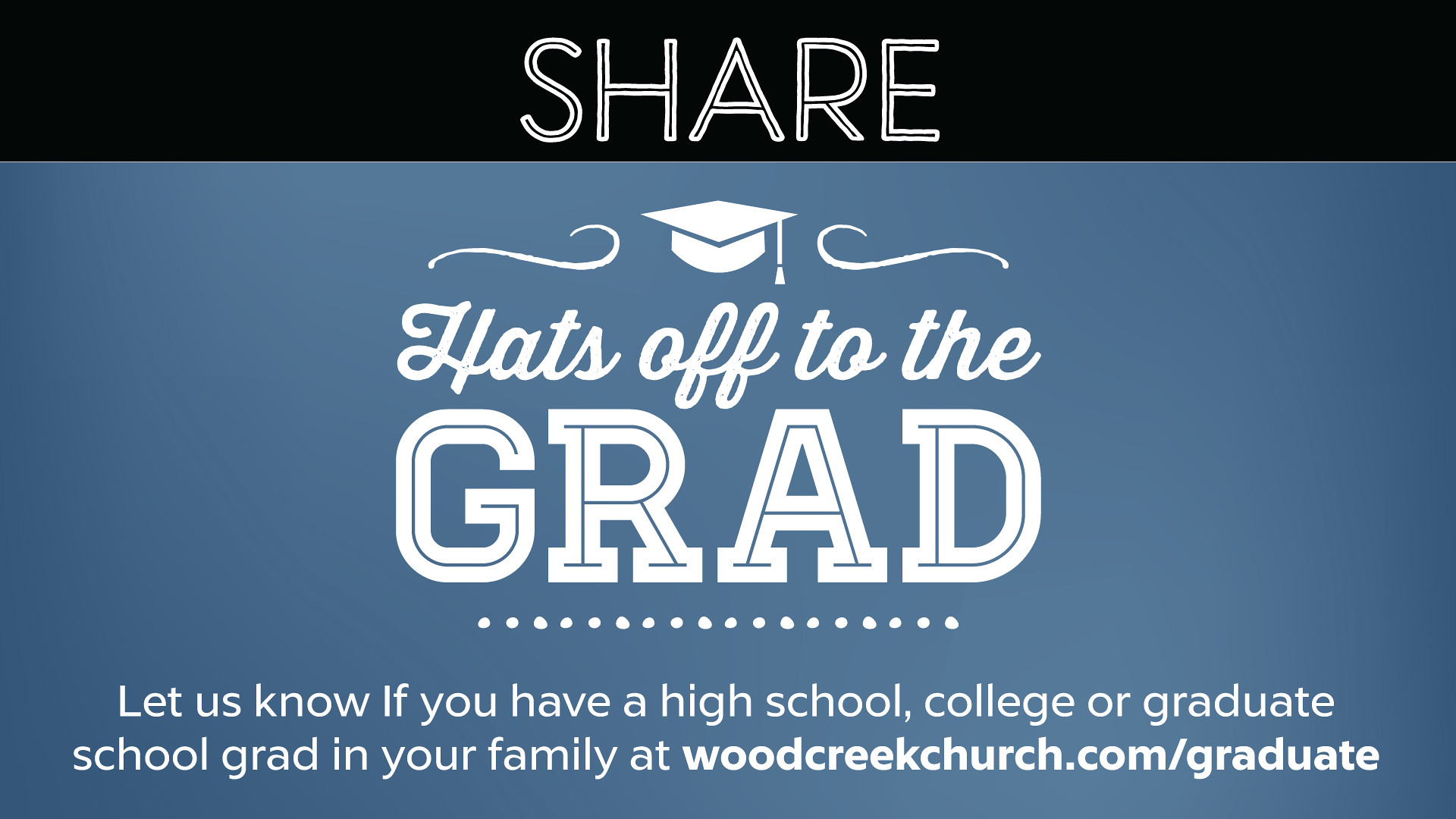The image is a promotional flyer with a predominantly blue background and key text elements in white. At the top, a black horizontal bar spans the width of the flyer, featuring the word "SHARE" in uppercase white letters. Below this, the blue background outlines the primary message: "Hats off to the grad," with a graduation cap icon above the text and a dotted white line beneath it. The bottom section of the flyer provides further information, reading, "Let us know if you have a high school, college, or graduate school grad in your family at woodcreekchurch.com/graduate."